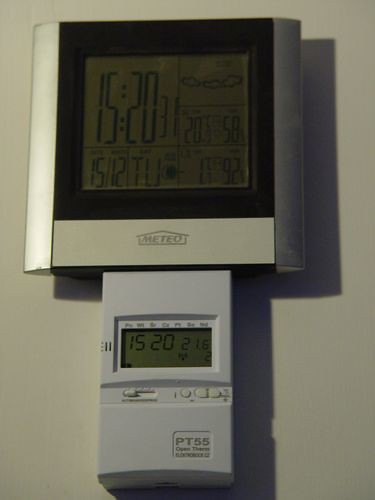The photo features two control boxes mounted against a pristine white wall. The larger box at the top displays a time of 15:20:31 in military format and includes additional numbers to its right. An image of clouds, possibly indicative of weather data, is depicted in the upper right corner, suggesting it is a product from the company Meteo. The top box is bordered in black with a white trim, containing a digital screen at its center.

Directly below, the smaller control box shows a time of 15:20 and an additional figure of 21.5. This unit, labeled PT 55, features knobs and buttons for making various adjustments. Both boxes cast a soft gray shadow against the white background, highlighting the light source illuminating them. The lower box is entirely white, except for its central digital display screen.